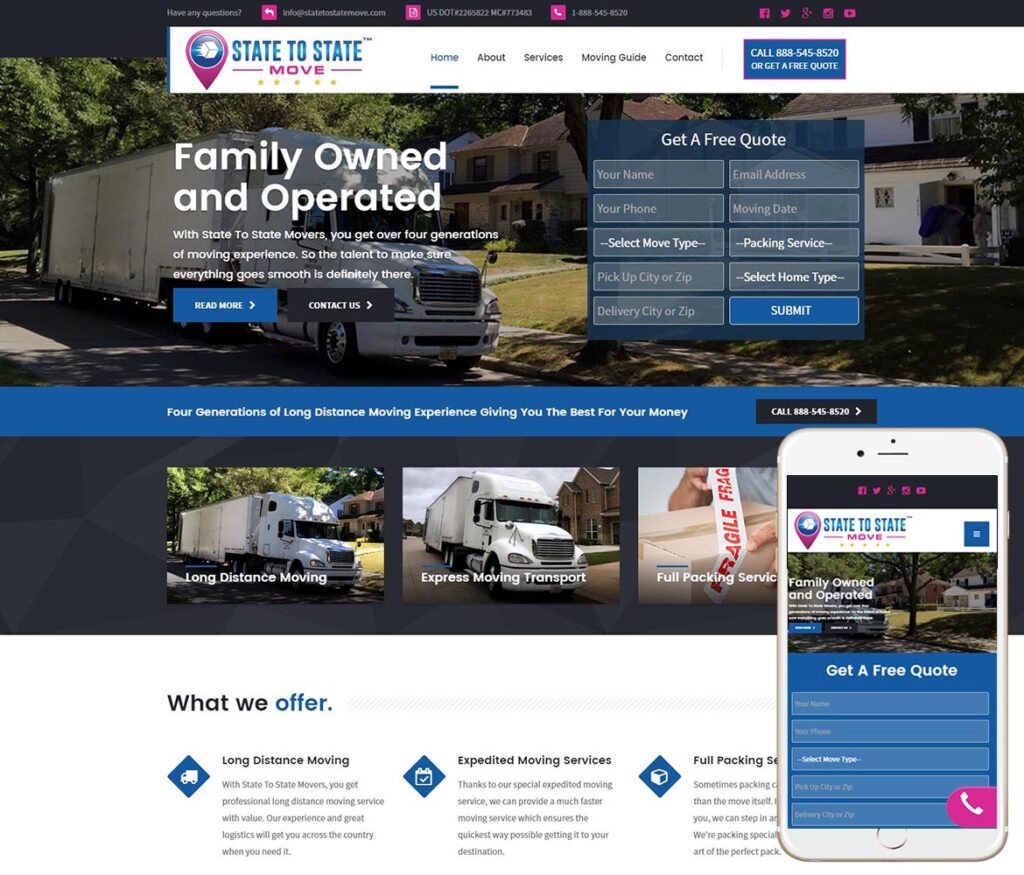The image is a detailed website screenshot from a moving company. At the top of the page, there is a navigation menu featuring options such as "State-to-State Move," "Home About Services," "Moving Guide," and "Contact." The "Home" tab is prominently highlighted in blue, suggesting the current page. The other menu options are displayed in black. Additionally, the page includes a contact number, 885-545-8520, and a prompt to get a free quote.

To emphasize the company's attributes, the page states "Family Owned and Operated." It features a scenic picture of a typical suburban neighborhood, with several homes and a moving truck parked in front of one of the houses, likely symbolizing the company's operational activities.

There are interactive buttons on the page, such as "Read More" displayed in a blue rectangle with white text and "Contact Us" shown in a gray rectangle with white text. Another section encourages potential clients to get a free quote by filling out a form that requests details like your name, email address, phone number, moving date, and various specifics related to the move, such as move type, packing service, pickup city or ZIP, delivery city or ZIP, and home type. All input fields are light gray, with the "Submit" button in blue.

The website also outlines the services offered by the company, including "Long Distance Moving," "Expedited Moving Services," and "Full Packing Services."